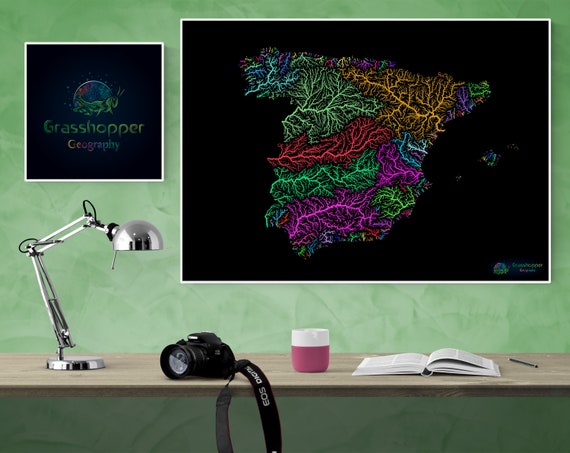The photograph captures a wooden desk against a green-gradient wall, where the green intensifies at the upper corners and lightens as it descends. On the left side of the desk, a flexible, silver desk lamp reminiscent of the Pixar lamp is visible. Right beneath the lamp, a traditional black camera with a strap is neatly placed. Beside the camera, there is a white and purple (or pink) coffee mug, followed by an open book with white pages. A pen lies horizontally to the right of the open book.

In the background, adorning the wall, there are two distinct artworks. On the left, a small black square with a white outline features a grasshopper in front of a globe, accompanied by the text "Grasshopper Geography." To the right, a larger rectangular piece with a white border showcases an abstract, colorful design with hues of greens, oranges, reds, purples, and blues, resembling divided mountain peaks. The scene is depicted in a landscape orientation and conveys a well-organized, artistic workspace.